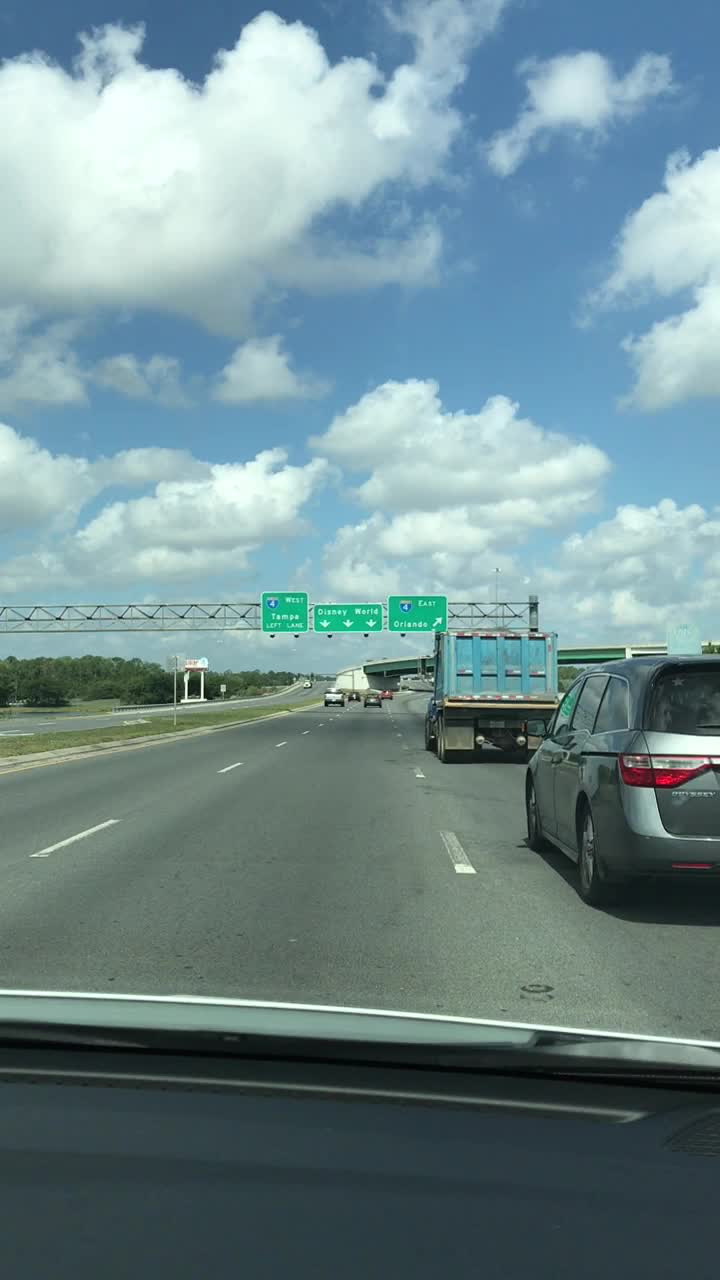This photograph, likely a still from a dash cam, captures a vibrant scene through the windshield of a car driving in the middle lane of a four-lane highway under a bright blue sky dotted with fluffy white clouds. The road is busy with a variety of vehicles, including a gray minivan and a blue work truck to the right, and a silver hatchback and a dump truck further ahead in the right lane. The left lanes have cars that are much farther ahead. The road is bordered by a grassy shoulder on the right and a green grass median. Above the road, three green traffic signs with white lettering on a metal bar indicate directions to Disney World and Tampa, although the text is too distant to read clearly. Trees line the horizon, completing the picturesque scene.